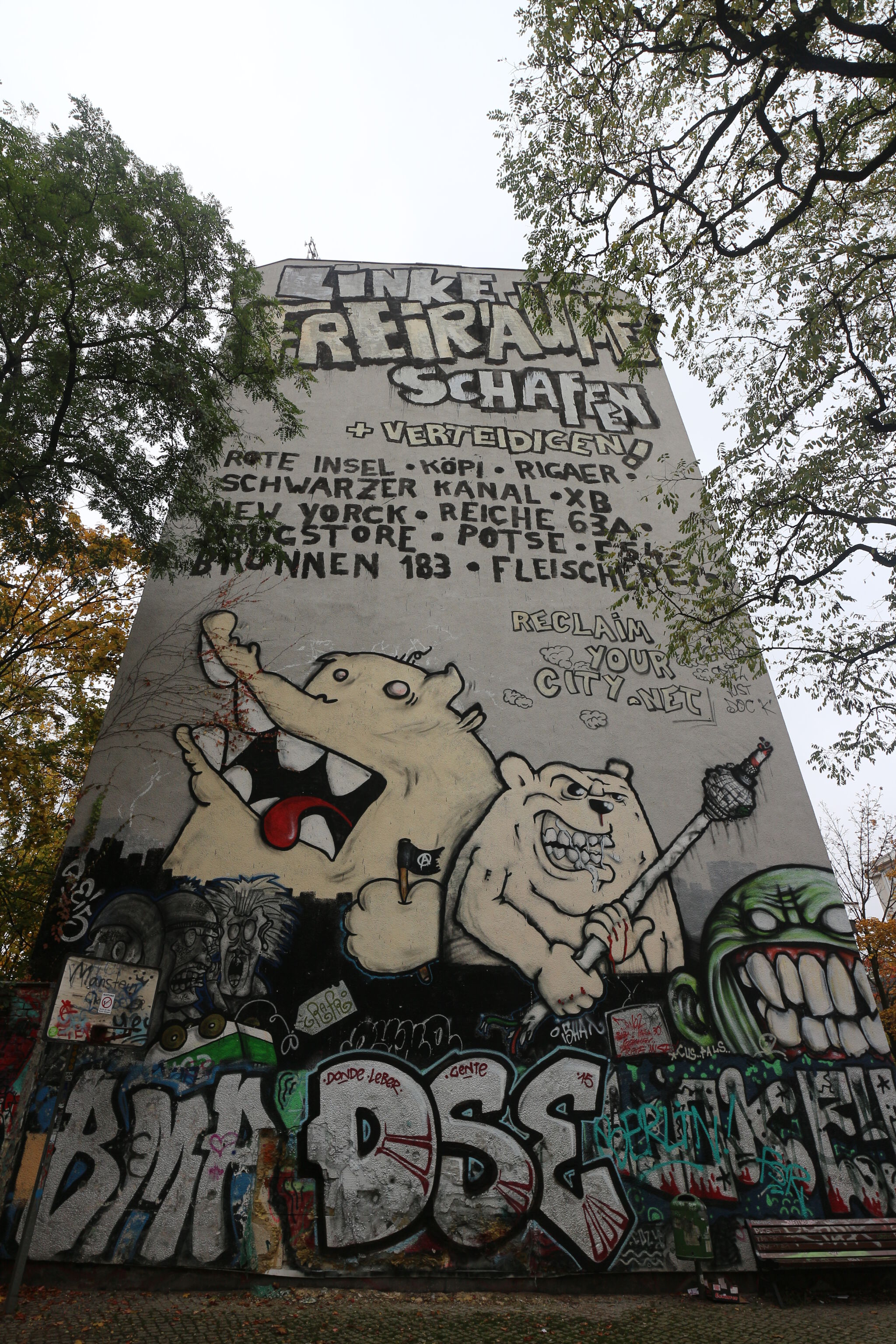The photograph captures a tall, narrow cement wall of a building, likely taken outside during the daytime. The wall is gray and heavily adorned with various graffiti. At the top, prominent graffiti text appears in different languages, potentially including German. Notable words include "LINKE," "FREIR’AUME," "SCHAFEN," "BERT’EID’GEN," "WROTEINCELL.COPEE.RIGAER," and "SCHWARZERCANAL.XB." Further down, the text reads "BRUNIN183," "FLEISHL," and "RECLAIMYOURCITY.NET." Beneath this array of text, graffiti depicts two rabid animals—a pig holding an anarchy flag and a bear wielding a bar. Additionally, there is an illustration of a green round head with white eyes and large white teeth in the lower right corner, alongside white-lettered graffiti such as "BMR" and "DSE."

The wall stands beside tall trees, and a park bench is situated at the bottom right of the scene, adding a sense of place and scale to the graffiti-covered structure.